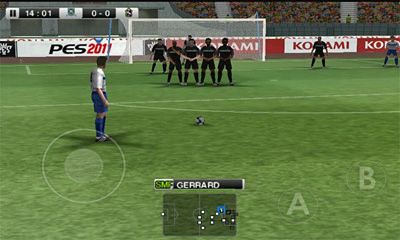This detailed video game screenshot captures an intense soccer match on a lush green field, centered around a player named Gerard, whose position on the team is indicated on a small map at the bottom of the image. Dressed in a white shirt, blue shorts, and blue socks, Gerard is poised mid-field, ready to make a critical play. The scene is set with a soccer goal visible in the distance, guarded by a cluster of players in black uniforms, comprising approximately half a dozen individuals. Additional players stand strategically positioned off to the side. Surrounding the field, a vibrant crowd fills the bleachers, adding to the high-stakes atmosphere of the game. The background prominently features branding from "PES 2011" and "Konami," accentuating the game's realistic environment. To the right of the map, there are noteworthy icons marked with a capital 'A' and 'B', enhancing the gaming interface. The scoreboard is located at the top left, though its details aren't fully captured in the image. The field itself is crisply demarcated with sport-specific lines, including a notable half-circle, emphasizing the layout's authenticity.